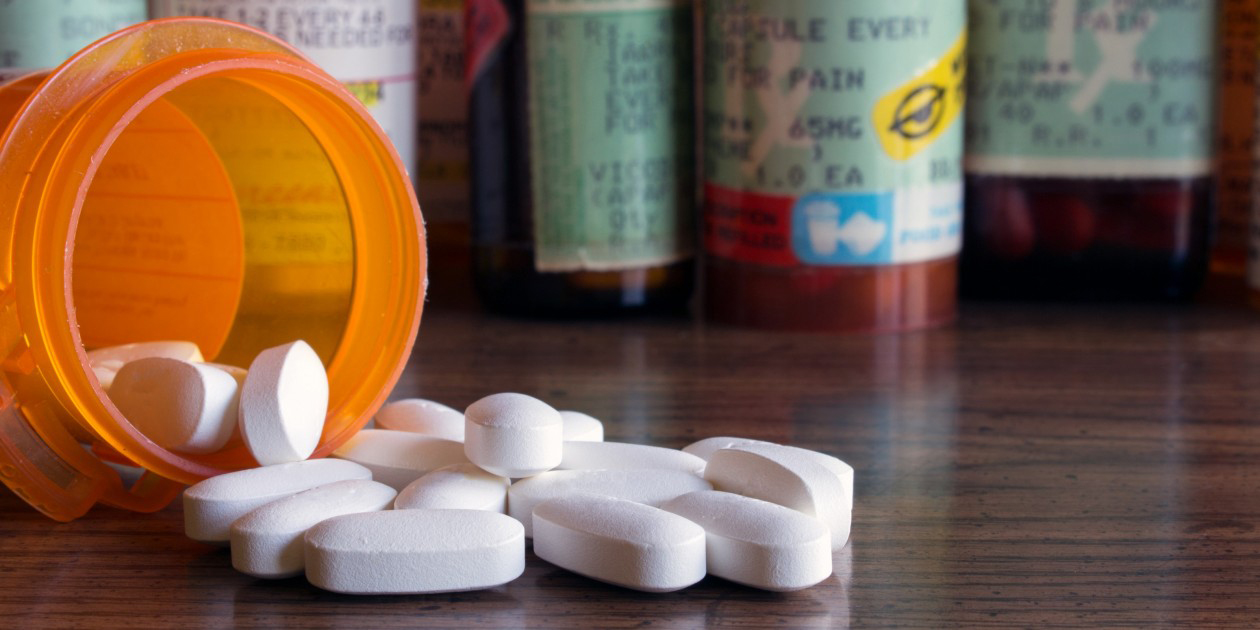The photograph features several white capsule-shaped pills scattered in a small pile on a dark brown wooden tabletop. An orange, slightly see-through pill bottle lies tipped over on the left side of the image, with more pills visible inside, giving the impression they recently spilled out. Approximately ten pills can be seen on the surface. Behind the spilled pills, a variety of prescription medication bottles of different sizes and colors are positioned, though most labels are blurry and difficult to read. One bottle distinctly has a teal label mentioning "pain" and indicates a dosage of 65 milligrams. Another label features a yellow sticker with an image resembling a drowsy eye, marked with a circle and a line through a half-black dot, symbolizing drowsiness. The scene suggests the need for caution, as the pills are not secured, highlighting potential safety concerns.